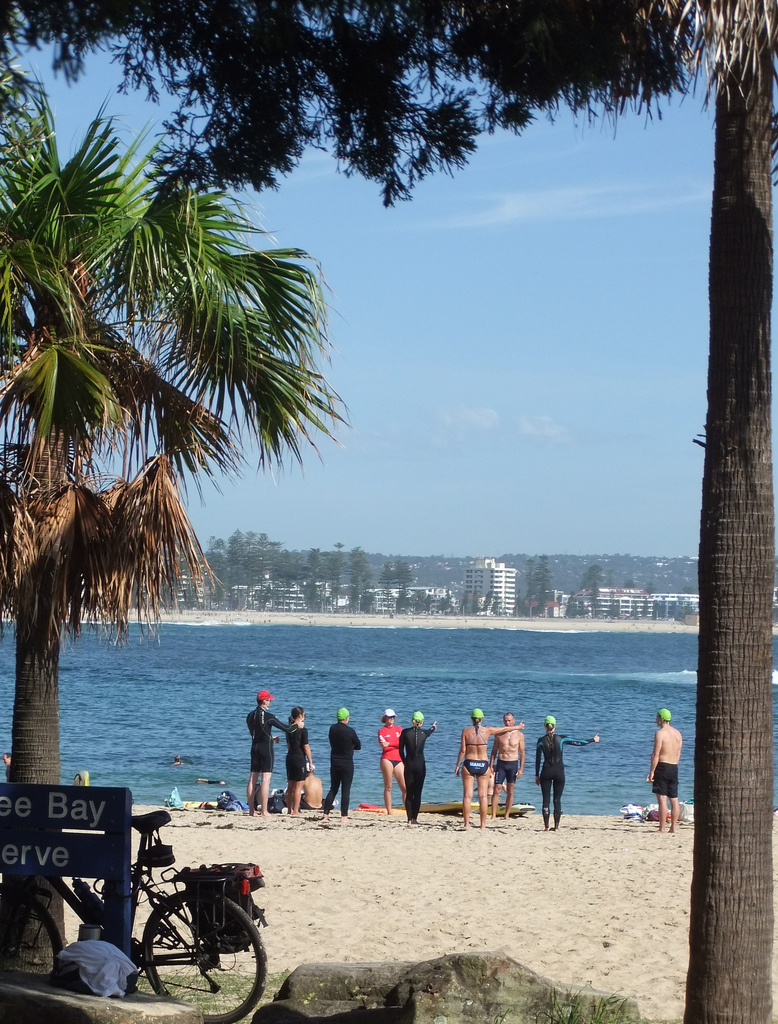In this photograph, a group of people is gathered on a sandy beach, framed on either side by large palm trees with both green and brown fronds. The participants, who appear to be preparing for an educational surfing session, are standing with their arms outstretched, possibly stretching or getting ready for a dive into the water. Wearing a mix of full-body wetsuits and bathing suits, most of them don neon green swimming caps for easy identification in the water. Several surfboards are scattered on the beach, emphasizing the surfing activity. A sign that partially reads "Bay Reserve" is visible on the left side of the image, indicating the location. Behind this sign, a bike park can be seen. The scene transitions from the sandy beach to a beautiful blue ocean and then to a distant shoreline dotted with buildings. The sky above forms a serene backdrop to the lively scene below.